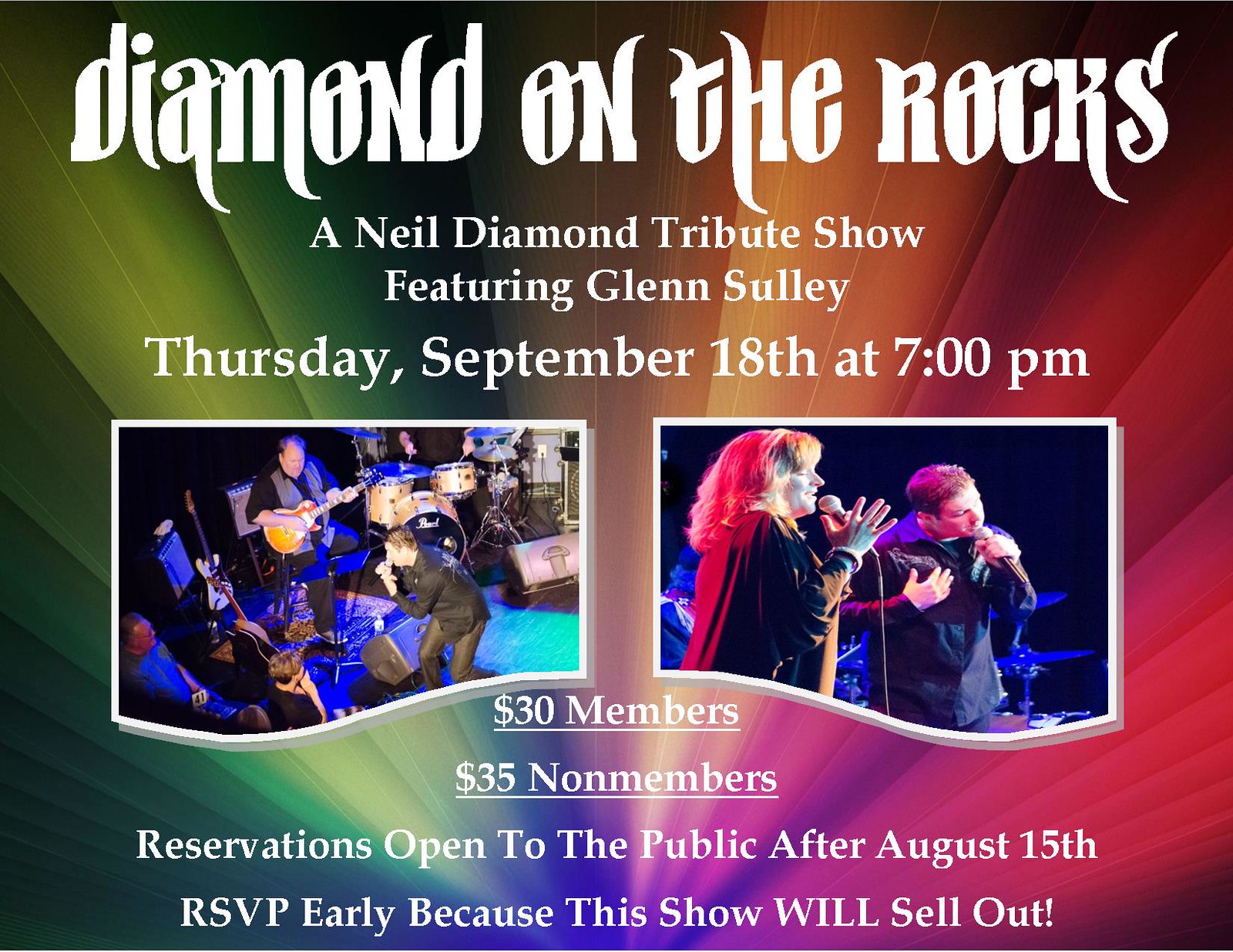This poster is for a musical performance titled "Diamond on the Rocks," a Neil Diamond tribute show featuring Glenn Sully. The background is a vibrant, rainbow-hued design with shades of green, red, orange, and other colors arranged in a pattern reminiscent of flowering leaves or flames shooting upwards. In the center, the poster features two photographs: the left photo depicts a three-member band with a drummer, a guitarist, and a vocalist, while the right photo shows a man and a woman singing into microphones. The top of the poster boasts the show's title, "Diamond on the Rocks," in a fancy font, followed by plain text that reads, "A Neil Diamond Tribute Show Featuring Glenn Sully." Below this, the event details are clearly stated: "Thursday, September 18th at 7 p.m." The bottom of the poster includes ticket pricing information, stating "$30 for members, $35 for non-members," both underlined, and a note that "Reservations open to the public after August 15th," along with a warning to "RSVP early because this show will sell out." The overall design appears to be a digitally created print, incorporating real photos seamlessly into the colorful, text-rich background.